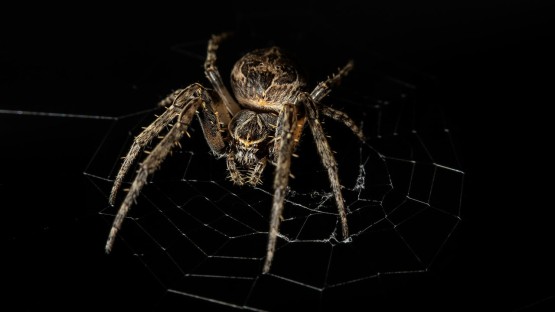In this highly detailed photograph, a large spider dominates the frame with the intricate details of its body expertly captured. Set against a pitch-black background, the spider appears on a nearly invisible, faintly discernible web, arranged in a circular formation and showing a break in the bottom right corner. The spider, predominantly brown and tan with hints of orange, stands poised at the center of the web. Its eight legs are clearly visible, with a bristly, spiky texture – six legs are grounded while two are raised, as if the spider is reaching towards the observer. The spider's abdomen features black spots, contrasting with its lighter body and furry jawline. The creature faces slightly to the left, giving the impression of looking directly into the camera, creating a haunting and intense atmosphere. The overall composition highlights the spider’s potential predatory patience in its dark setting.